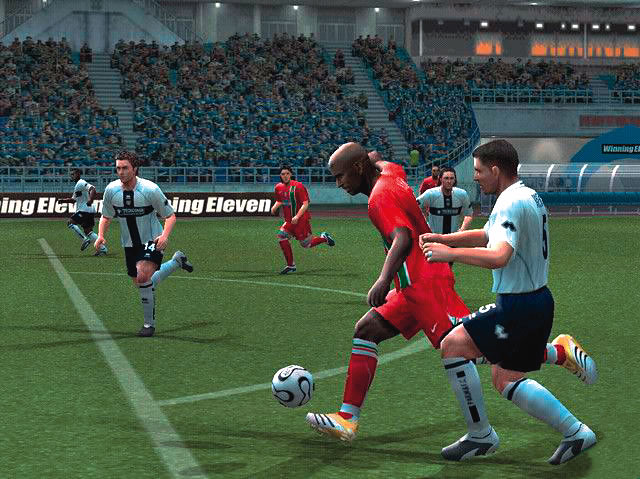This image captures a dynamic moment in a soccer video game, likely from the FIFA series, where two teams are engaged in an intense match. The field is bustling with players dressed in distinct uniforms; the team in red is facing off against the team in white. The focus is on a player in a red uniform who is executing a powerful kick, with an opponent in white nearby, closely contesting the move. In the background, other players from both teams are seen running towards the action, adding to the sense of urgency and competition. The stadium is packed with spectators whose presence is represented by pixelated blobs, suggesting a packed arena filled with cheering fans. The image's quality diminishes with distance, becoming noticeably pixelated towards the back, highlighting the limitations of the video game's graphics at that depth.